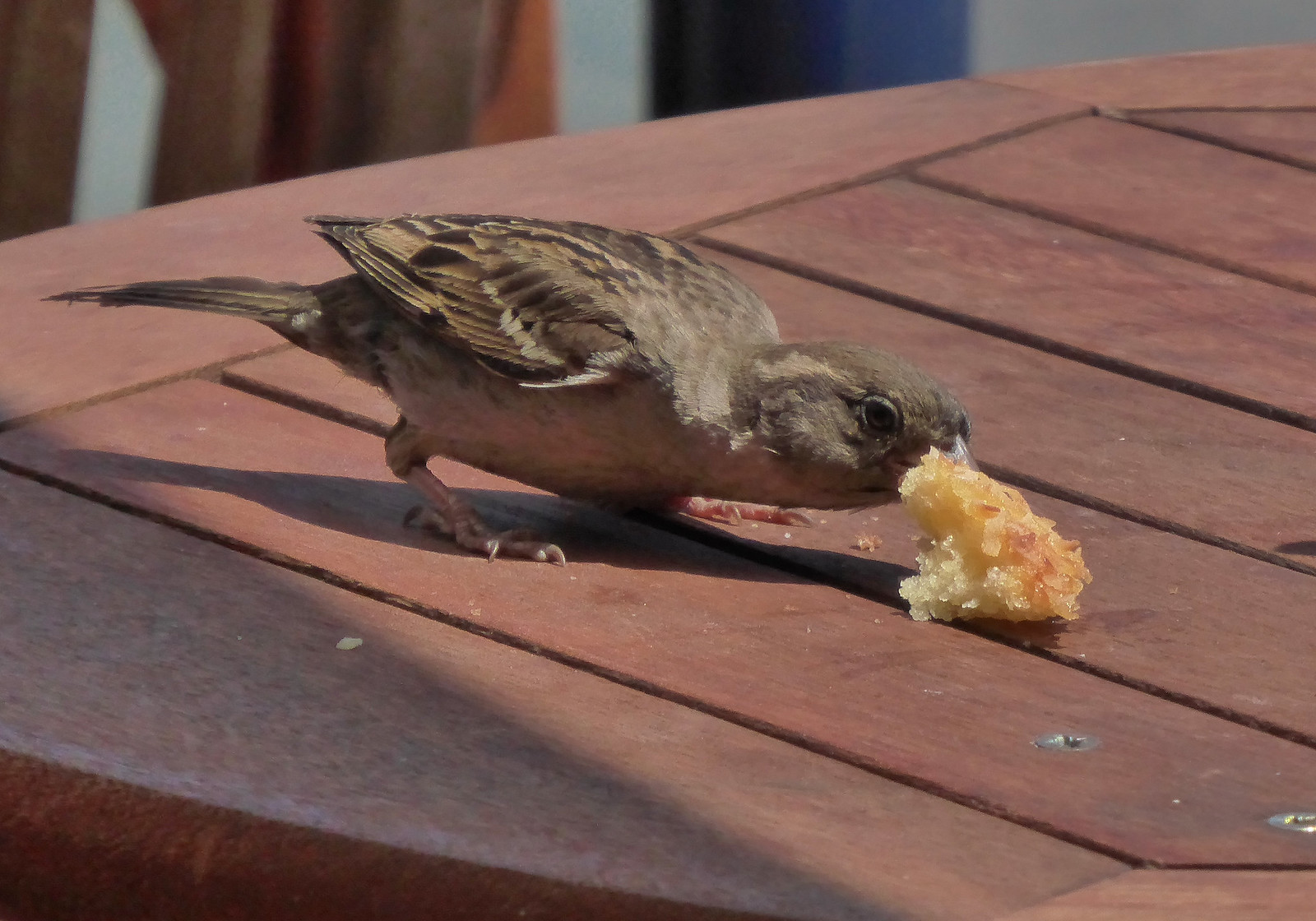In this outdoor photograph, a brown sparrow with lighter tan feathers and distinctive pink legs is captured in the center of the frame, hunched over and nibbling on a yellow, starchy-looking morsel resembling a piece of cake or possibly a hash brown. The food item, which appears fried or greasy, lies on a worn, red picnic table characterized by boards oriented from the upper left to the lower right corner. There's noticeable staining on the table, including what looks like bird droppings in the lower right corner. The setting seems to be outside near a building, possibly on a boardwalk or patio, with the table edges suggesting an umbrella table. The bird's activity has left marks on the table where it has slid the food back and forth.